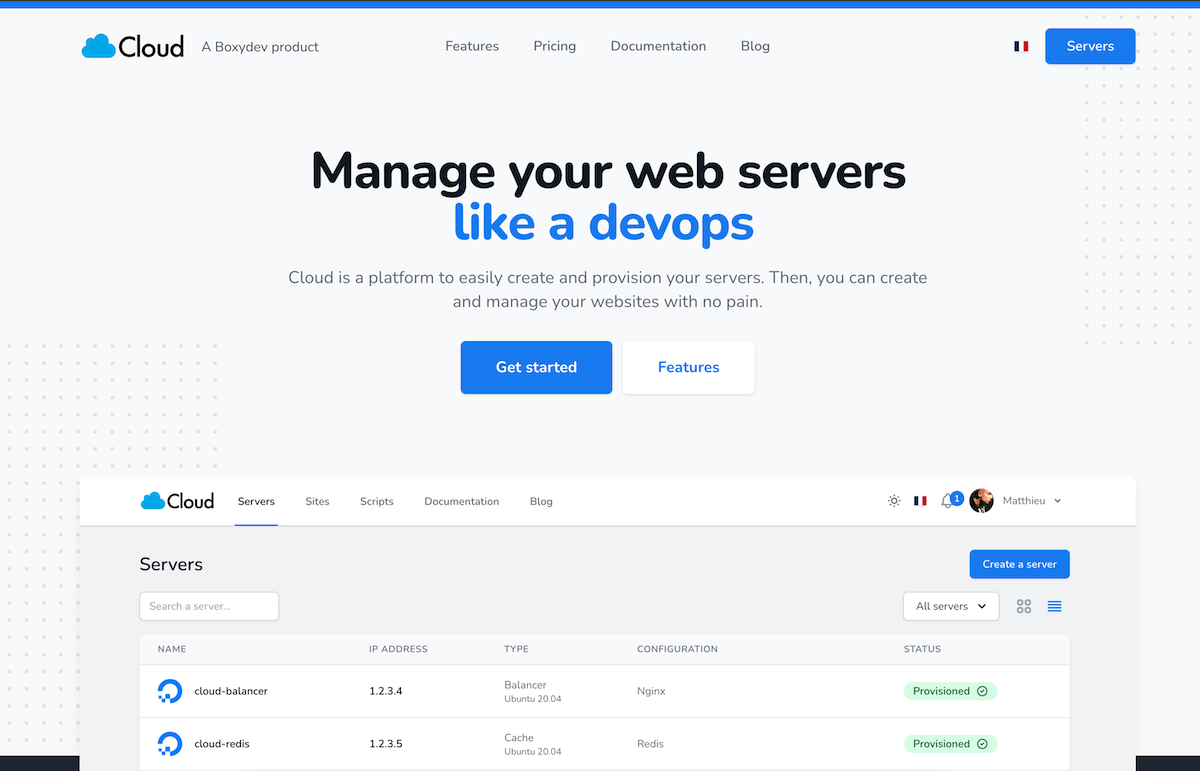The image features a gray background accented with a thin blue border at the top. In the upper left corner, there's a blue cloud icon accompanied by the bold black text "Cloud." Below this, it reads "A Boxy Dev Product." Centrally, the text "Features, Pricing, Documentation, Blog" is displayed prominently. The upper right corner showcases a flag icon next to the word "Servers" in white, accompanied by a blue button.

Further down, the caption "Manage your web servers like a DevOps" is boldly presented. Underneath, it describes the service: "Cloud is a platform to easily create and provision your servers. Create and manage your websites with no pain." Two prominent buttons are visible here: a blue button with white text that says "Get Started," and a white button with blue text that says "Features."

At the bottom, the image depicts an interface of the service in use. The same blue cloud icon and the word "Cloud" appear again, this time followed by the options "Servers, Sites, Scripts, Documentation, Blog." On the far right, there's a profile icon. The interface section lists options such as "Server, Select a Server, Cloud Balancer, and Cloud Redis." Additionally, it features a section where users can "Create a Server," along with details for servers including "Name, IP Address, Type, Configuration, and Status."